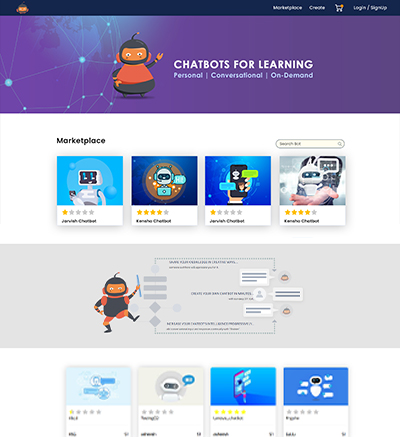This screenshot depicts an unknown website displaying various AI chatbot courses or creations. In the top left corner, there is a blurred shopping cart icon, a login/sign-up option, and a marketplace link. Dominating the top of the screen is a vibrant banner featuring an animated robot in an orange shirt against a purple background. This banner advertises "Chat Boxes for Learning" and "Chat Bots for Learning," emphasizing their personal, conversational, and on-demand nature.

Beneath this, a white banner lists four different marketplace options, each represented by a chatbot. The text descriptions are indistinct, but the ratings are visible: the first option has received one star, the second four stars, the third one star, and the fourth four stars.

Following this, a gray banner displays an image of a robot balancing on one foot beside an unreadable flow chart. Below this, four additional chatbot options are presented with varying ratings: the first has half a star, the second has no stars, the third has five stars, and the fourth again has no stars.